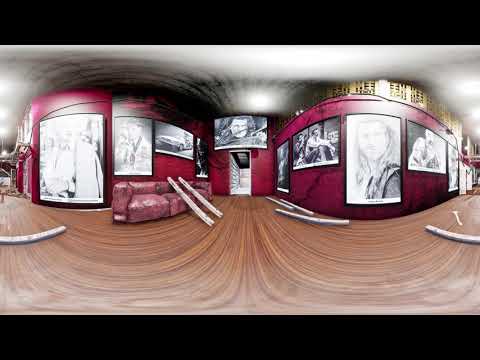The image depicts a highly distorted and warped interior of a building, where the floor and walls curve in an exaggerated manner, creating a surreal, cylindrical effect. The floor is made of light brown, tan wood, bending along with the image. The walls are predominantly maroon or burgundy, adorned with numerous black-and-white photographs and sketches in black frames. These images vary in size and shape, showing individual portraits and grouped figures. A white doorway located centrally in the background adds a point of depth to the warped perspective, with an all-white room visible behind it.

In front of the wall on the left side of the image is a lighter maroon couch, upon which rolled-up posters or sketches are leaning. Additional similar posters are scattered on the floor around the couch. There is a noticeable gold trim where the wall meets the ceiling on the right-hand side. The overall scene is chaotic, with plywood and various objects strewn across the floor, enhancing the sense of disarray caused by the warped visual effect. Additional hues observed in the image include dark purple, fuchsia, and hints of light pink, gold, black, and white. Some text, possibly in a different language, is visible but not legible.